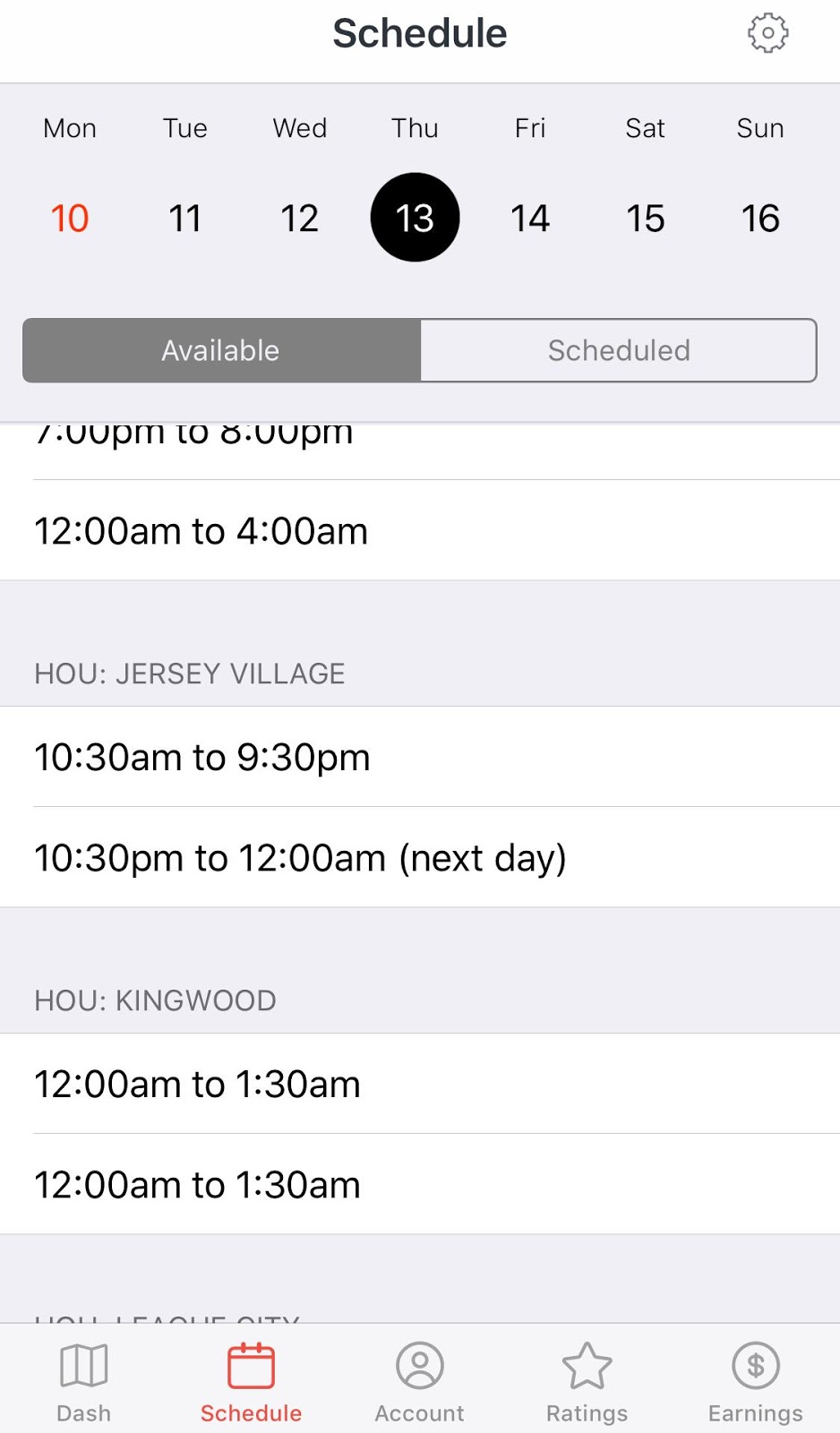The image is a screen capture of a phone interface, characterized by its size and shape. The top of the display lacks typical indicators such as battery life or the current time, beginning instead with a plain white background. Centered prominently in the middle, the word "Schedule" appears in bold black lettering. To the right of this title is a gray gear icon, indicating settings.

Beneath the title, there’s a gray box displaying the days of the week in three-letter abbreviations (Mon, Tue, Wed, Thu, Fri, Sat, Sun). Alongside the days are corresponding dates, with Monday in red and Sunday marked as the 16th. Notably, Thursday is highlighted with a bold black circle encompassing white text.

Below this, the interface presents two options in colored boxes: “Available” and “Scheduled.” The "Available" option is dark with lighter text, while the "Scheduled" option is white with gray text.

Further down, specific hour-long slots are listed, spanning various times:
- 7 p.m. to 8 p.m.
- 12 a.m. to 4 a.m.

The next section lists time slots for specific locations:
- Houston Jersey Village: 10:30 a.m. to 9:30 p.m. or 10:30 p.m. to 12:00 a.m. the next day.
- Houston Kingwood: 12:00 a.m. to 1:30 a.m.

Each location's timeframe offers choices, presumably for scheduling purposes.